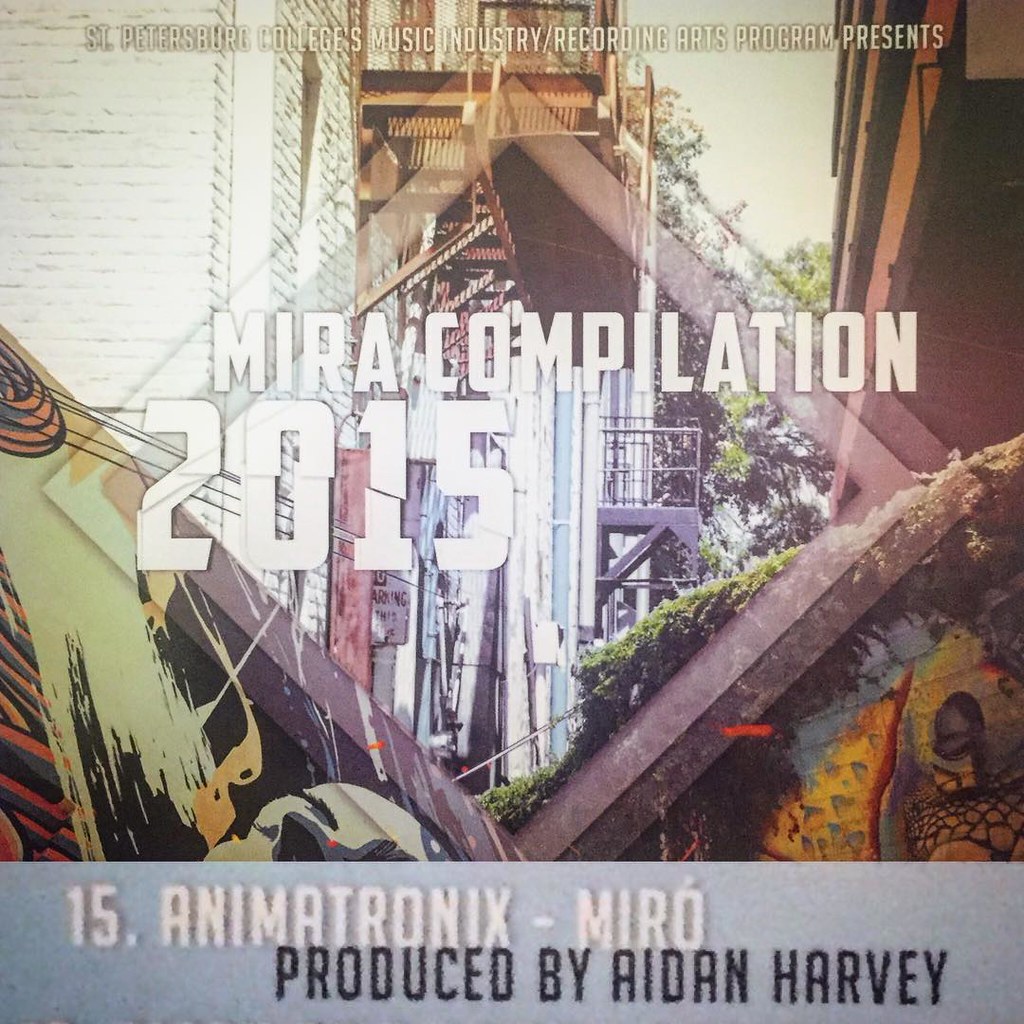The image in question appears to be an album cover or flyer from 2015, associated with an event by the St. Petersburg College Music Industry/Recording Arts Program. The setting is an outdoor scene, likely in an alleyway between buildings featuring rusty fire escapes and steps, with some visible parts of a park or courtyard adorned with graffiti murals. The background includes trees, suggesting a sunny day.

In the foreground, there's a collection of randomly colored boards and debris, including a small shed with grass on the roof and large boards leaning against it. Prominently displayed in a diamond shape in the center of the image, there is white text that reads "MIRA Compilation 2015". At the top, in white letters, it says, "St. Petersburg College's Music Industry/Recording Arts Program Presents." Below the main title, the text credits the producer, Agent Harvey. The border at the bottom of the image features the label "Almatronics-MIRA" with additional white and black text detailing production credits.